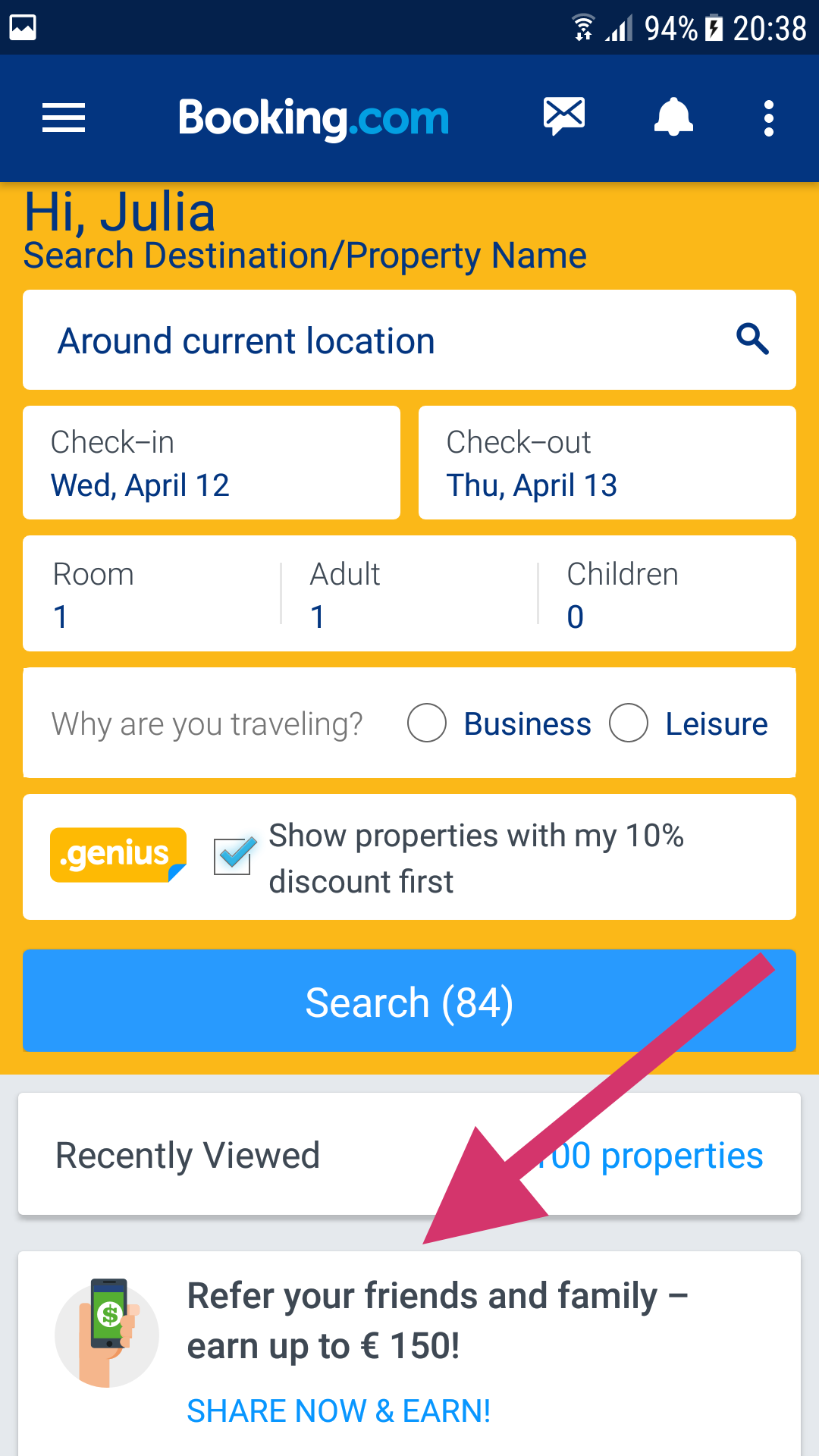Here’s a detailed caption for the image based on your description:

---

This mobile screenshot showcases the booking.com website interface, encapsulated within a sleek design. At the top, a prominent blue header displays the booking.com logo centrally, flanked by a menu icon on the left and an envelope, alert, and three dots icon on the right. Dominating the next section, a gold background warmly greets the user with "Hi Julia," followed by a prompt to search for a destination or property name, indicating Julia is logged into her account.

Directly beneath, a user-friendly search bar allows for location-based searches, displaying options for checking in and out on Wednesday, April 12th, and Thursday, April 13th, respectively. A subsequent selection bar provides easy adjustments for the number of rooms, adults, and children, currently set to one room and one adult. Travel purpose options for business or leisure are available but remain unselected.

Highlighted within this layout is the Genius logo, accompanied by a checkmark option to filter properties eligible for a 10% discount. Just below, a prominent blue search bar invites the user to initiate the search process. At the bottom of the interface, the user’s recently viewed properties are on the left, with total property count to the right. Superimposed with a red arrow, an edited note points to a referral opportunity, “Refer your friends and family and earn up to 150."

---

This caption provides a comprehensive breakdown of the image, ensuring clarity and context for anyone viewing it.